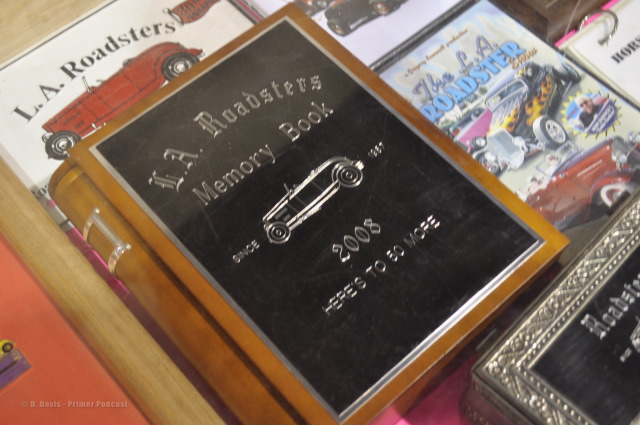The image showcases a carefully arranged collection of memorabilia centered around a prominent brown memory book with a black cover and silver-framed plaque. This book, titled "L.A. Roadsters Memory Book: Since 1957, Here's to 50 More," is placed front and center and is turned slightly counterclockwise. Also visible is a sign featuring a red hot rod car and the words "L.A. Roadsters." To the right, there is another book dedicated to roadsters, displaying various images of hot rod cars, aptly titled "Life of a Roadster." Among the items is a silver-framed container inscribed with the word "Roadster." All these pieces are laid out flat on a surface, creating a nostalgic and visually appealing spread of L.A. Roadsters memorabilia.